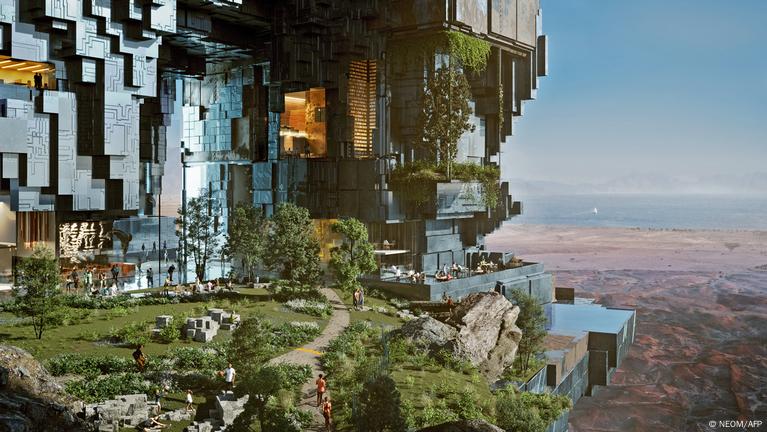This rectangular image, approximately six inches wide and three inches high, captures a stunningly detailed scene. Dominating the left two-thirds of the picture is an enormous, futuristic mansion elegantly perched on a natural cliffside, far above the ground. Made of large panels that resemble metal with circuitry, this grand building features various facades and a balcony extending over a barren valley below. The lower portion reveals a meticulously landscaped garden walkway adorned with green grass, vibrant flowers, hedges, and trees, with humans leisurely strolling along the path. The right part of the image showcases a serene landscape, featuring a dry, brown hillside that transitions into a picturesque beach and a glistening water body, all under a vivid blue sky. Overlooking this scene are also amber-colored lights visible through the mansion's windows, adding a warm ambiance to the futuristic setting. In the lower right-hand corner, the photo is marked with a white copyright symbol followed by "Neo M / AFP".